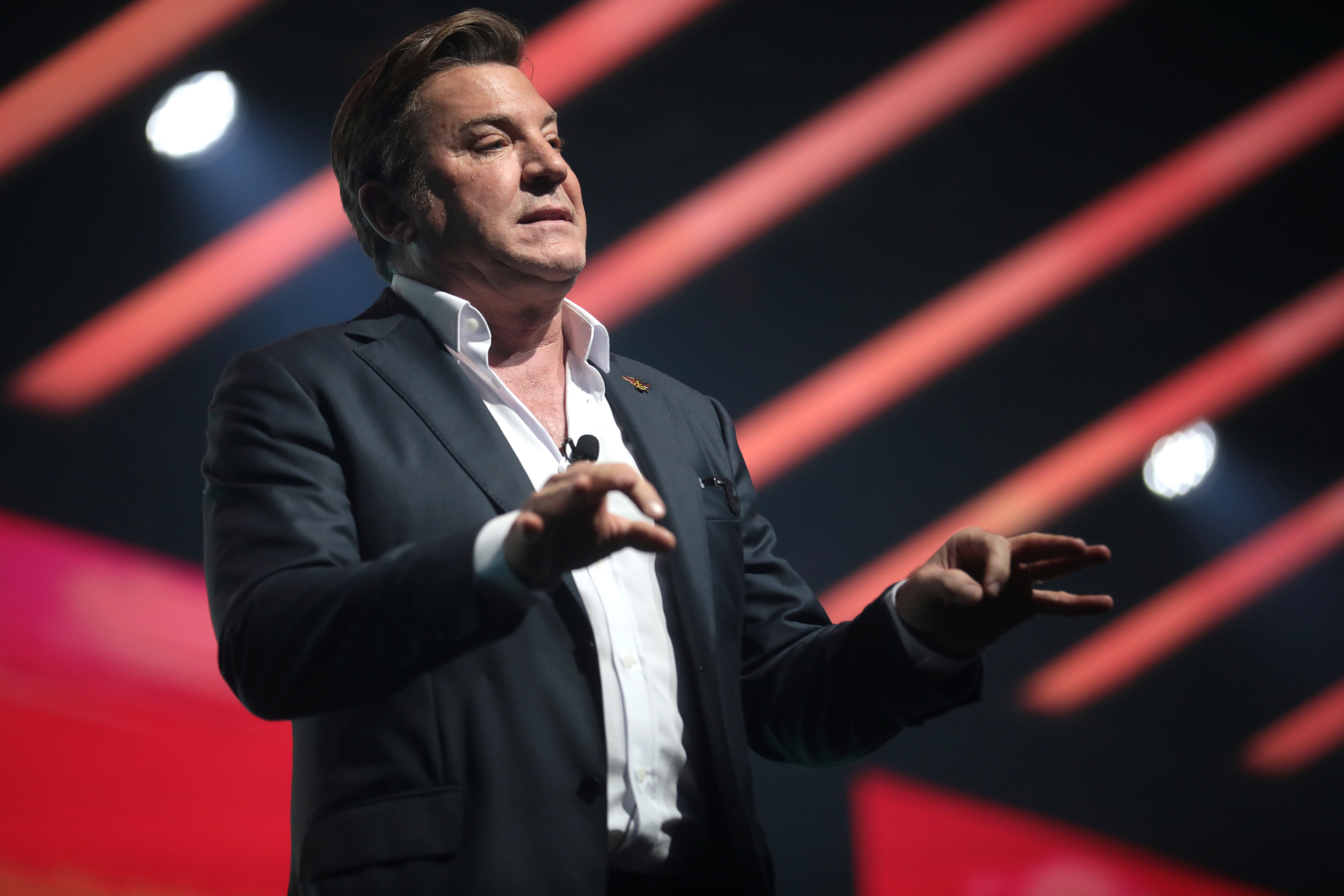The photograph captures a middle-aged man, likely in his 40s, giving a presentation. He stands to the left of center with only his upper body visible, framed in a landscape orientation shot. The man has short brown hair and wears a black business coat over a white button-up shirt, where the top three buttons are undone, creating a V-neck appearance. A small pin adorns the right lapel of his coat, and a black round microphone is clipped to his shirt near the bottom of the opening. He gestures with his hands in front of him, fingers forming circles as if he is emphasizing a point.

The background features a wall that is predominantly red, which could be formed by banners or screens, though the precise details are blurry due to the photograph's focus. Above him is a black roof with multiple red support beams and large, white spotlights that shine downwards.